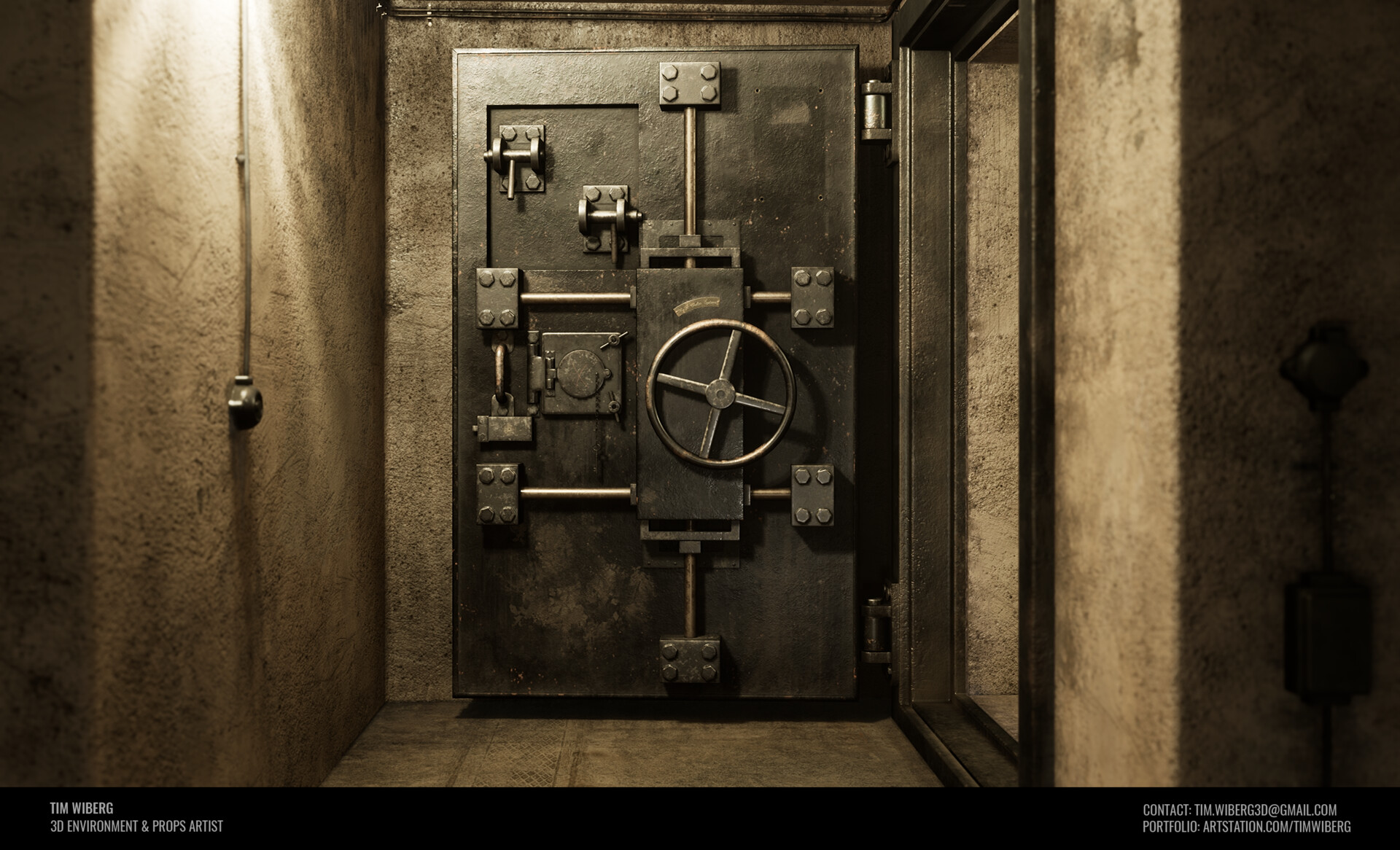This image likely shows a digital illustration or photograph of a bunker or vault door, centered within the frame. The door is robust, metallic, and grey, with a round, four-spoked wheel at its center, likely used to trigger its complex locking mechanism, which includes various rectangular parts and four circular elements connected by pipes. The door is open to the right, revealing a vault-like interior. The surrounding walls, distressed and painted in shades of brown, frame the scene, while the floor is also a matching beige or brown. A light source is visible on the left side of the hallway, illuminating the sparse, cavernous space. White text is written at the bottom on either side of the image, enhancing the industrial atmosphere akin to a safety locker or high-security vault.